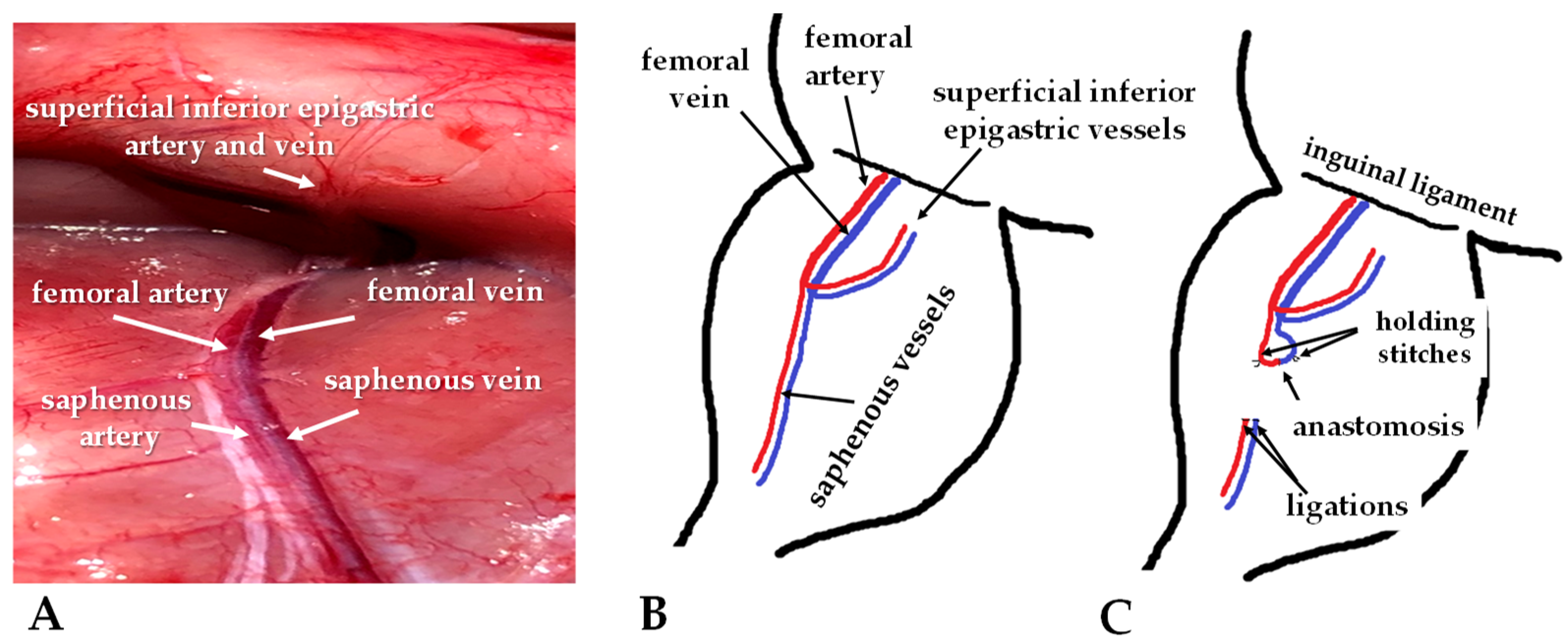The image is a detailed, three-part anatomical illustration labeled as sections A, B, and C. 

**Section A** features a full-color, photographic depiction of human flesh with a primary artery running vertically, identified at the top as the superficial inferior epigastric artery and vein. Labels point to various parts, naming the femoral artery, femoral vein, saphenous artery, and saphenous vein, with the arteries and veins clearly distinguished. 

**Section B** presents a line art sketch displaying the same vascular structures as in A—the femoral artery and vein, the saphenous vessels, and the superficial inferior epigastric vessels—illustrated with red and blue lines to differentiate arteries and veins.

**Section C** shows a line art diagram of the inguinal ligament, with labels indicating holding stitches, anastomosis, and ligations, suggesting a surgical context. This section focuses on the ligation and connection of the vessels around the inguinal ligament area.